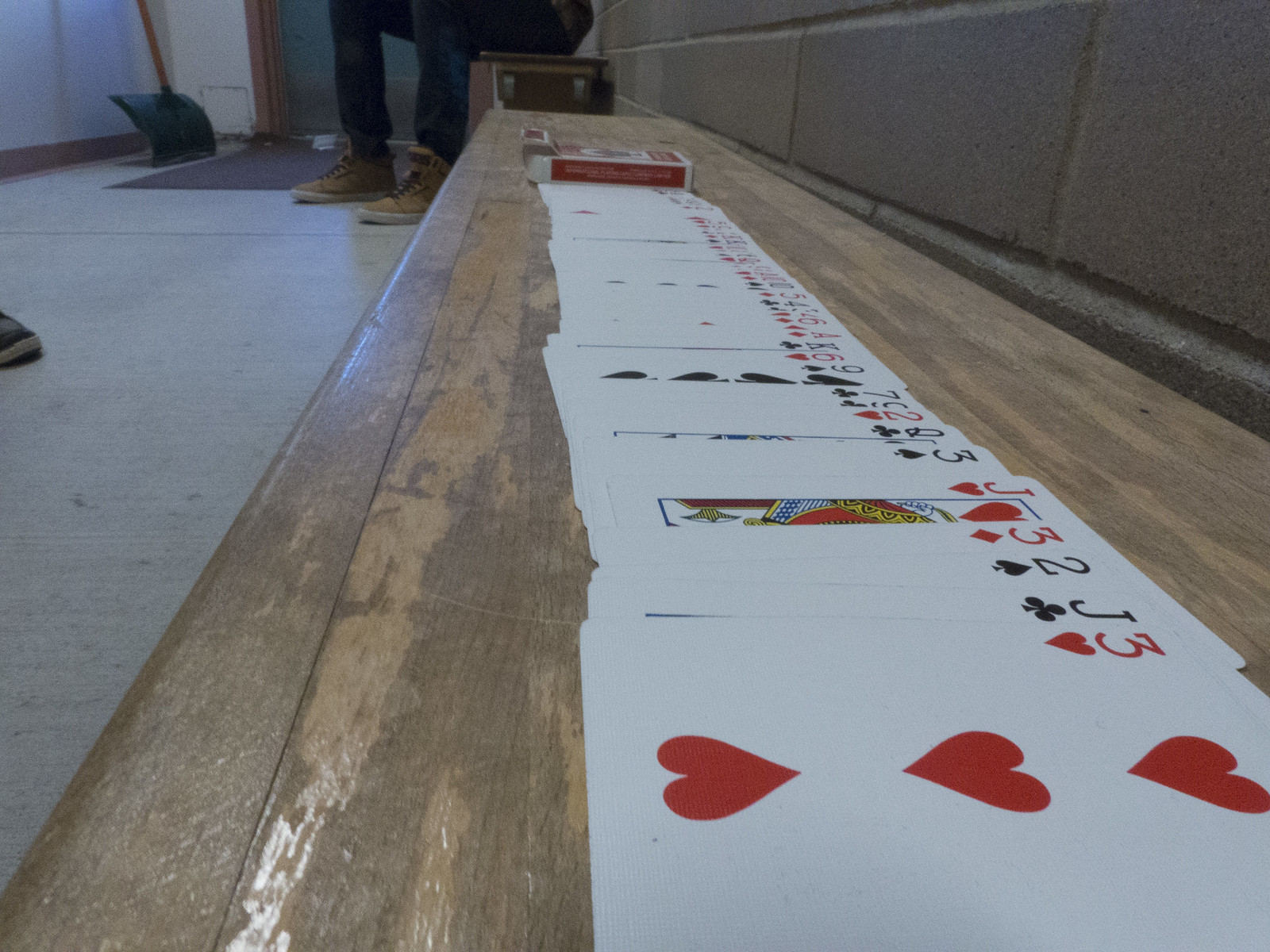In this portrait-oriented photograph, the primary focus is a close-up of a long wooden bench, which appears significantly weathered and worn. Spread out on the bench is a complete deck of standard playing cards, meticulously splayed face up to display every card in the deck, showcasing the reds for the hearts and diamonds, and the blacks for the spades and clubs. Next to the cards, there is the original box they came in, appearing quite old.

Behind the bench is a gray concrete block wall. The floor, which seems to be made of concrete as well, does not show much detail. The bench itself sits very low to the ground, almost just a step up from the floor level.

On the left-hand side of the image, there is a hint of a person's shoe, which is light tan in color. The person is wearing blue slacks. Behind them, to the left against the wall, there is a green-bladed snow shovel leaned against the wall. Also visible on the floor is a mat intended for wiping shoes and a dark green door with a heavily worn metal kick plate at its base.